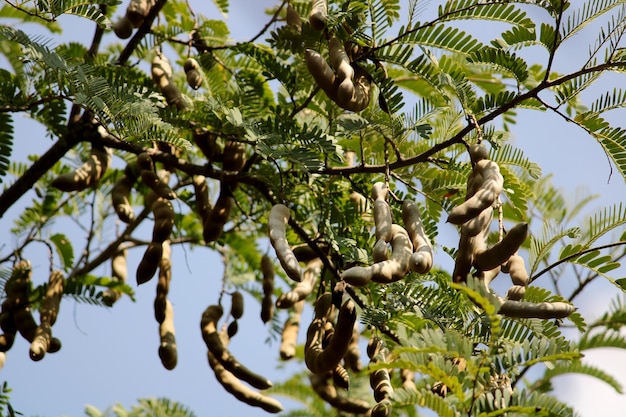The photograph captures an upward-looking view of a tree branch adorned with pods reminiscent of large, brown edamame. Around 20 nuts hang from the branch, which is surrounded by lush green leaves. The background reveals a partly cloudy blue sky with a hint of overcast, and a single cloud is visible in the bottom right corner. The tree itself bears a resemblance to a banana tree with its palm-like fronds, and the light brown pods hanging from the branches look ready for harvest.